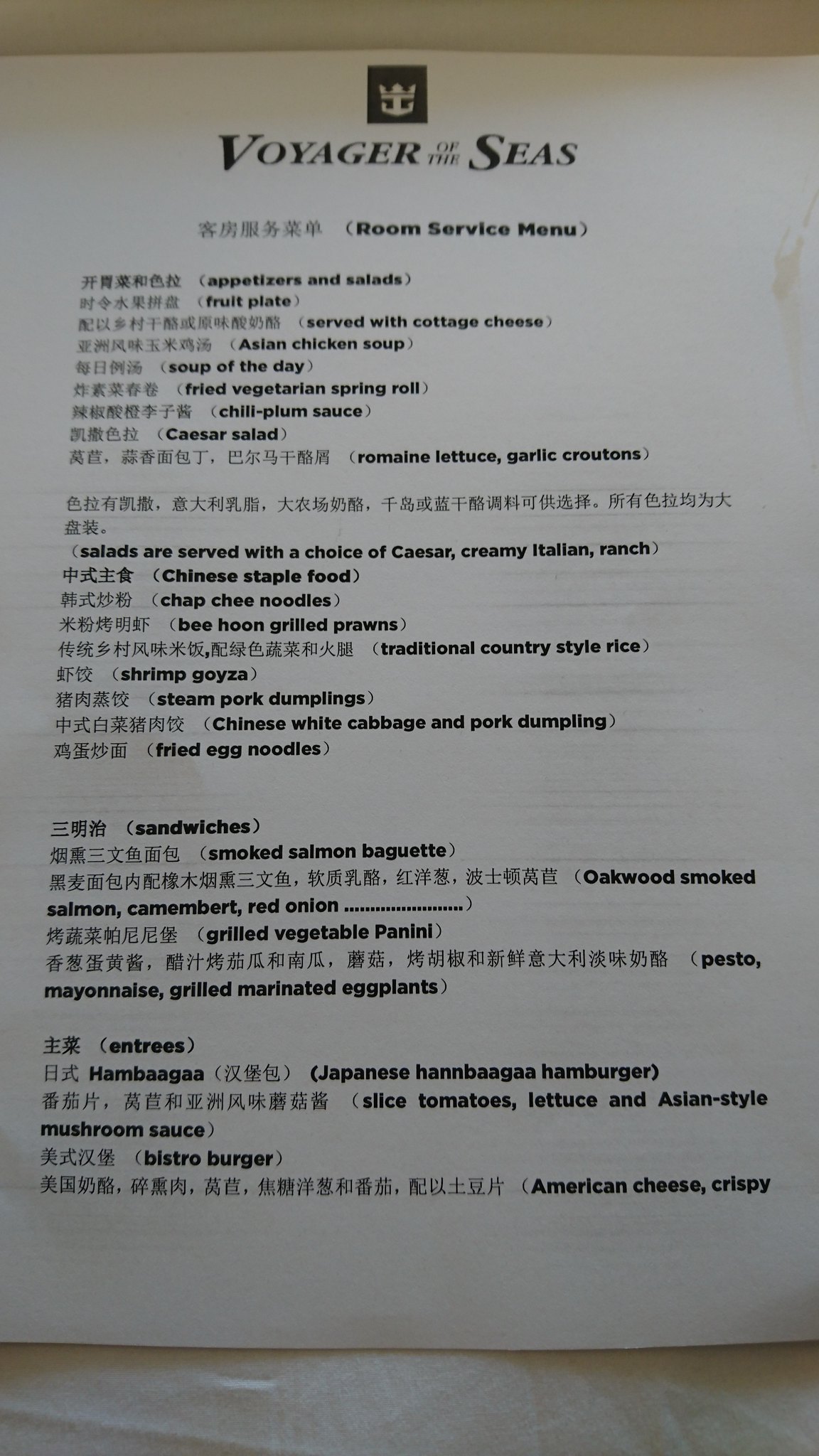The photo showcases a detailed room service menu from Voyager of the Seas, featuring a distinguished logo of a crown atop an anchor. The menu is primarily in Chinese with English annotations, offering an extensive selection of dishes across various categories. 

**Appetizers and Salads:**
- Fruit Plate served with Cottage Cheese
- Asian Chicken Soup
- Soup of the Day
- Fried Vegetarian Spring Roll with Chili Plum Sauce
- Caesar Salad with Romaine Lettuce and Garlic Croutons (Salads are served with a choice of Caesar, Creamy Italian, or Ranch dressing)

**Chinese Staples:**
- Chap Chi Noodles
- Bee Hoon
- Grilled Prawns
- Traditional Country Style Rice
- Shrimp Goyza
- Steamed Pork Dumplings
- Chinese White Cabbage and Pork Dumpling
- Fried Egg Noodles

**Sandwiches:**
- Smoked Salmon Baguette (Oakwood Smoked Salmon, Camembert, Red Onion)
- Grilled Vegetable Panini (Pesto, Mayonnaise, Grilled Marinated Eggplants)

**Burgers:**
- Japanese Hanbaga Hamburger (Sliced Tomatoes, Lettuce, Asian Style Mushroom Sauce)
- Bistro Burger (American Cheese, Crispy Onions)

The menu offers a diverse range of cuisines including traditional Chinese, Japanese, and Western-inspired dishes, appealing to a wide array of tastes.